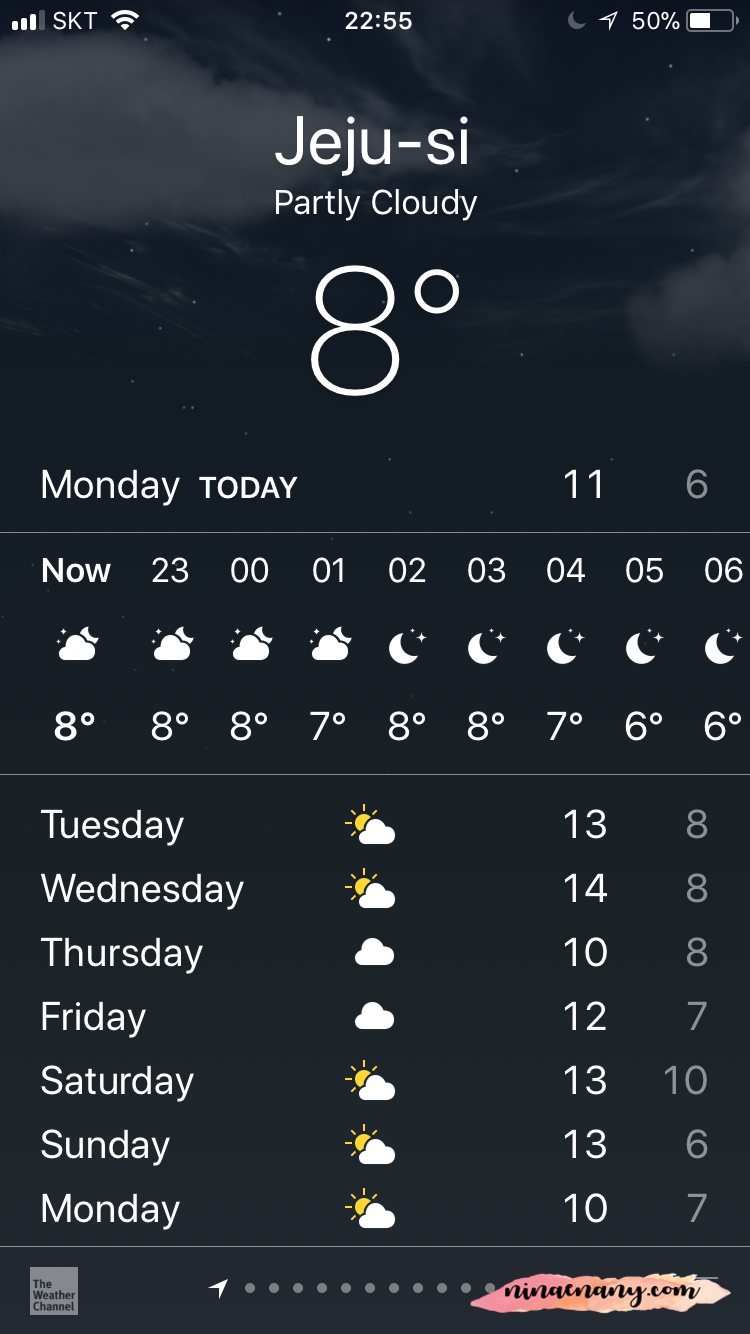The image is a screenshot of a weather application on a mobile device, displaying the forecast for Jeju-si. The background is a nighttime scene with a dark, starry sky and some clouds. At the top center, "Jeju-si" is prominently displayed, followed by the current weather condition, "Partly Cloudy," and a temperature of 8°C. Below this, the current day, "Monday," and the current time, displayed in a 24-hour format as "23:00," are shown. The hourly temperatures range from 8°C to 6°C.

Further down, a 7-day forecast for Tuesday through the following Monday is presented, with icons indicating mostly partly cloudy days, interspersed with a few cloudy ones. Each day's high and low temperatures are listed to the right. 

In the bottom left corner, the Weather Channel logo is visible, while a web address is displayed on a pink and peach-colored background on the bottom right.